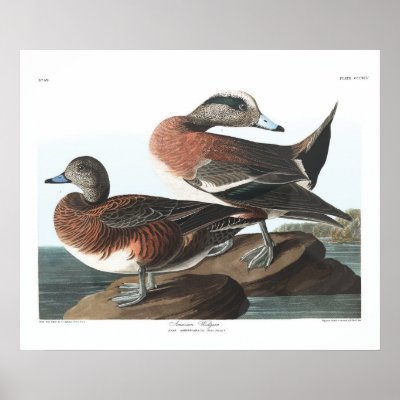This image presents a painting of two ducks perched on light brown rocks, overlooking a dark bluish-green body of water, likely a lake, with a stark white sky as the backdrop. The artwork itself is encased within a vertical rectangular frame, set against a gray background, with a white border. Text is indicated at the bottom of this border, although it remains unreadable due to its small size.

Focusing on the ducks, the one on the left, positioned foremost in the foreground, is shown in profile facing left. This duck exhibits brown and green feathers across its breast and wings, transitioning to white feathering on the belly and underside. The head is decorated with light gray and brown feathers, suggestive of a female duck, and it has a blue beak with a black tip, along with gray legs and feet.

The duck on the right, slightly larger and positioned higher up on the rocks, has its body facing left but has craned its neck at a 180-degree angle to face right, displaying what appears to be an expression of surprise. This duck, likely the male, boasts a white beak with a black tip and a distinctive streak of white feathering over the crest of its face, extending to a black streak over the eye and down the back of its neck. The head feathers present a mix of gray, brown, and black speckles. Its neck features light orange or red feathering that transitions into bright green, black, and white hues across its back and wings. The underbelly is adorned with white feathering, and the tail is slightly raised, revealing the white underbelly and black feathers at its base. Both ducks, with their intricate and colorful plumage, stand serenely on the rocks, adding a touch of liveliness to the tranquil lakeside scene.